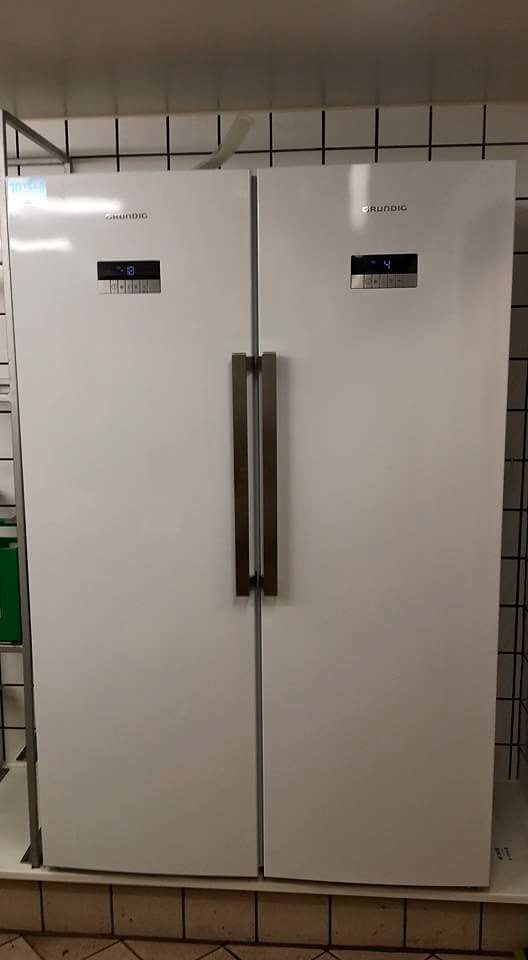This image features a sleek, white, double-door appliance, potentially a refrigerator, positioned against a white tile wall backdrop in an indoor setting. The refrigerator is tall, wide, and primarily white with vertical silver bar handles meeting centrally. Each door prominently displays the brand name "GroomDig" in small gray font near the top. Below the brand name, there is an illuminated black screen displaying a number, accompanied by several smaller, indistinguishable silver buttons likely for temperature control. The appliance appears to be situated on a slightly elevated white surface, underlining its possible use in a home, office, or medical environment. Light reflections highlight the appliance's polished silver elements, adding a touch of modernity and functionality.